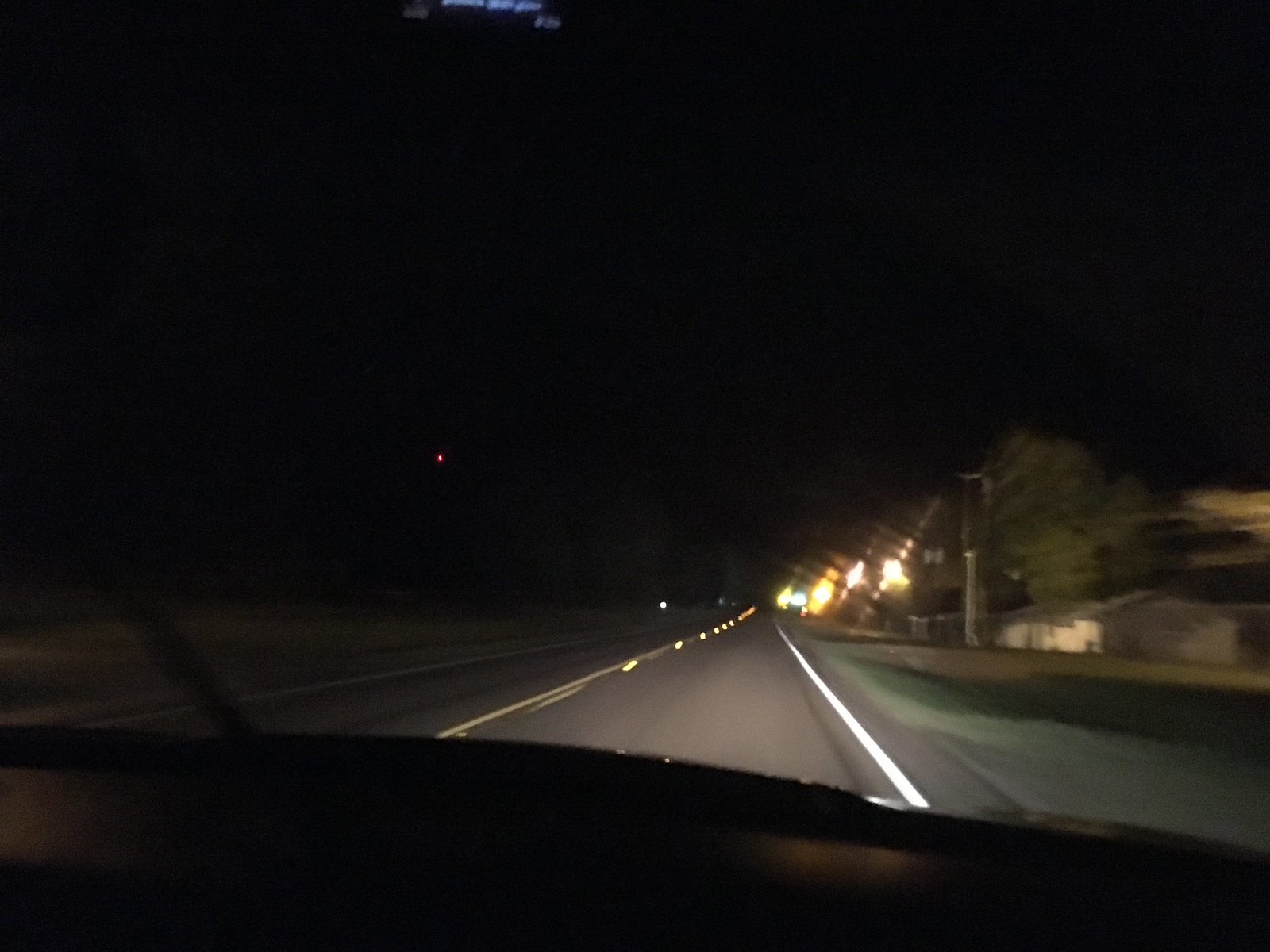The photograph captures a nighttime scene from the perspective of inside a moving vehicle. The image prominently features a two-lane road with a solid line on the left and a dashed line on the right, indicating the potential for passing. The dashboard and the windshield wipers of the car are visible, suggesting the picture was taken from the driver's or passenger's seat. The headlights cast a white glow on the road ahead, while the dark night sky forms a stark backdrop.

To the right of the road, the image reveals a blurry scene comprising what appear to be residential homes, some with porch lights, vaguely illuminated by nearby street lights. A tree is also discernible on this side. Off in the distance, additional street lights form a series of bright spots, potentially marking the boundary of a neighborhood or populated area. To the left, the scene is largely devoid of structures, appearing as open land with possibly a single distant light or star punctuating the horizon. The top of the image features some blue markings, suggesting the presence of a rearview mirror. Overall, the photograph encapsulates the quiet and somewhat eerie essence of night driving through a secluded road flanked by occasional signs of habitation.